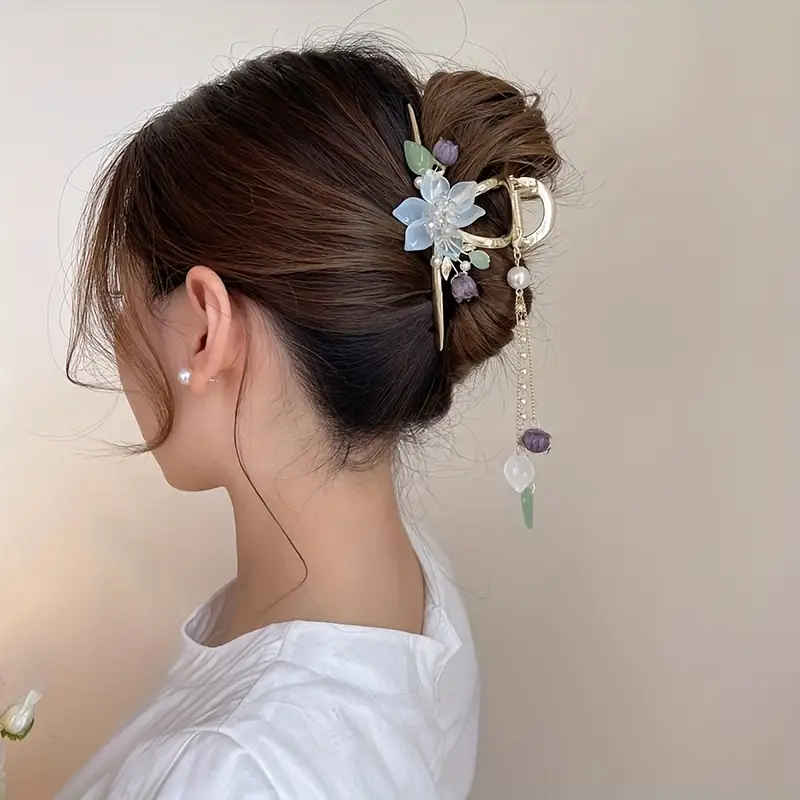In this image, we see a detailed view of the back and side of a woman's neck and face, set against a tan background. She is dressed in a simple white shirt and wears a single pearl earring. Her dark brown hair is styled in a twisted updo, secured by an ornate metallic gold hair clip. The clip itself is adorned with intricate light blue and purple glass flowers, as well as delicate green glass leaves. Adding to its elegance, a long trailing chain extends from the clip, featuring glass ornaments including pearl and purple beads, clear accents, and green, leaf-like glass pieces.